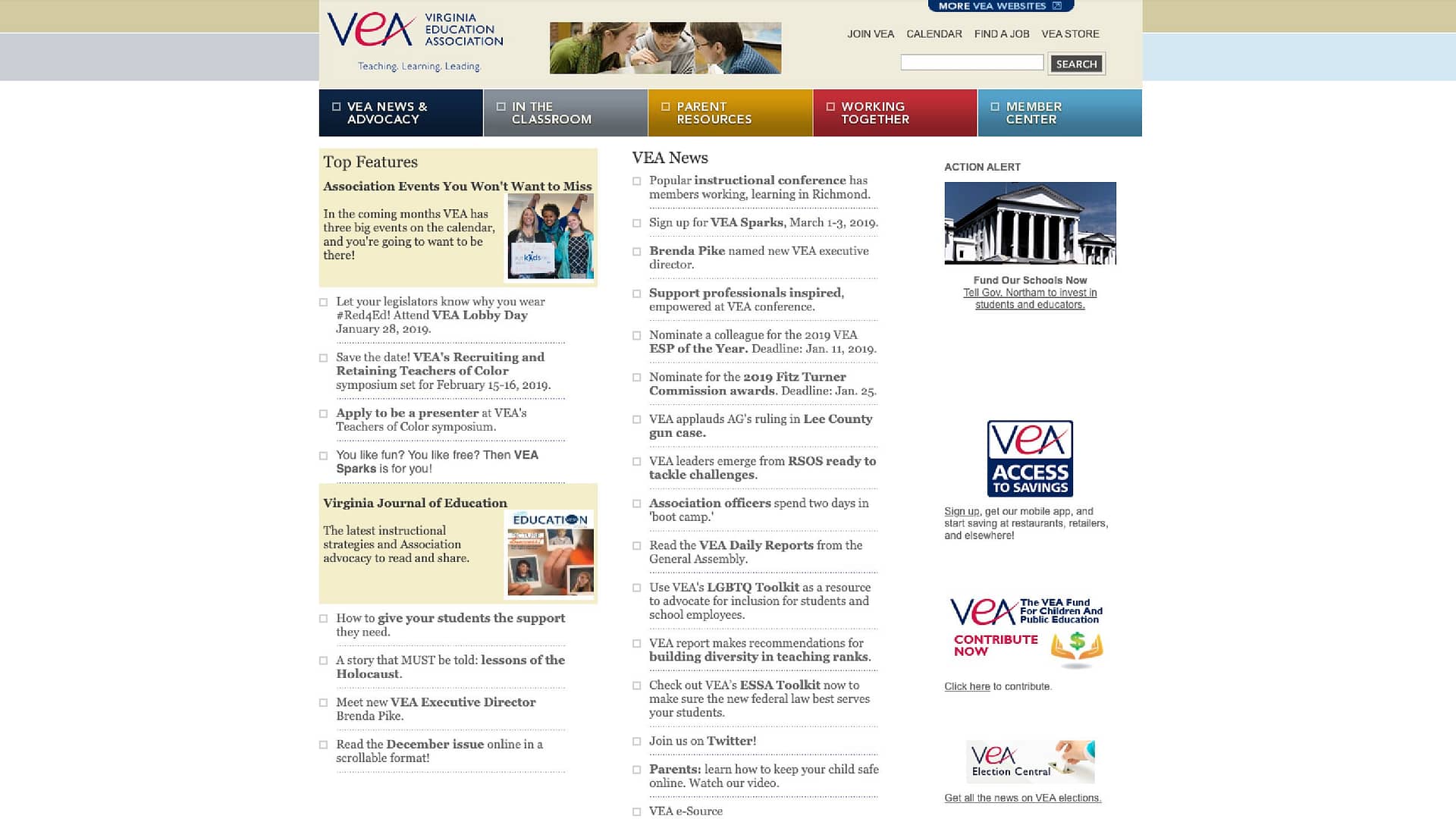The Virginia Education Association's website features a top section with a beige-colored background, showcasing a photo of three junior high students in a classroom setting. A search bar is conveniently located on the top right, accompanied by main navigation links such as "News and Advocacy," "In the Classroom," "Parent Resources," "Working Together," and "Member Center."

The page also includes several small and difficult-to-read news headlines. On the right side of the homepage, there's an "Action Alert" section advocating for school funding with the banner "Fund Our Schools Now." The main page features a white background with black text and numerous small links scattered throughout the page. Among these links are prompts to join VEA on Twitter and articles such as "VEA Applauds AC's Ruling in Lee County Gun Case." Another notable feature includes a photograph of students and a section promoting association events not to be missed. The "Virginia Journal of Education," akin to a magazine cover, also appears prominently among the various news articles that are presented, albeit in small, hard-to-read text.